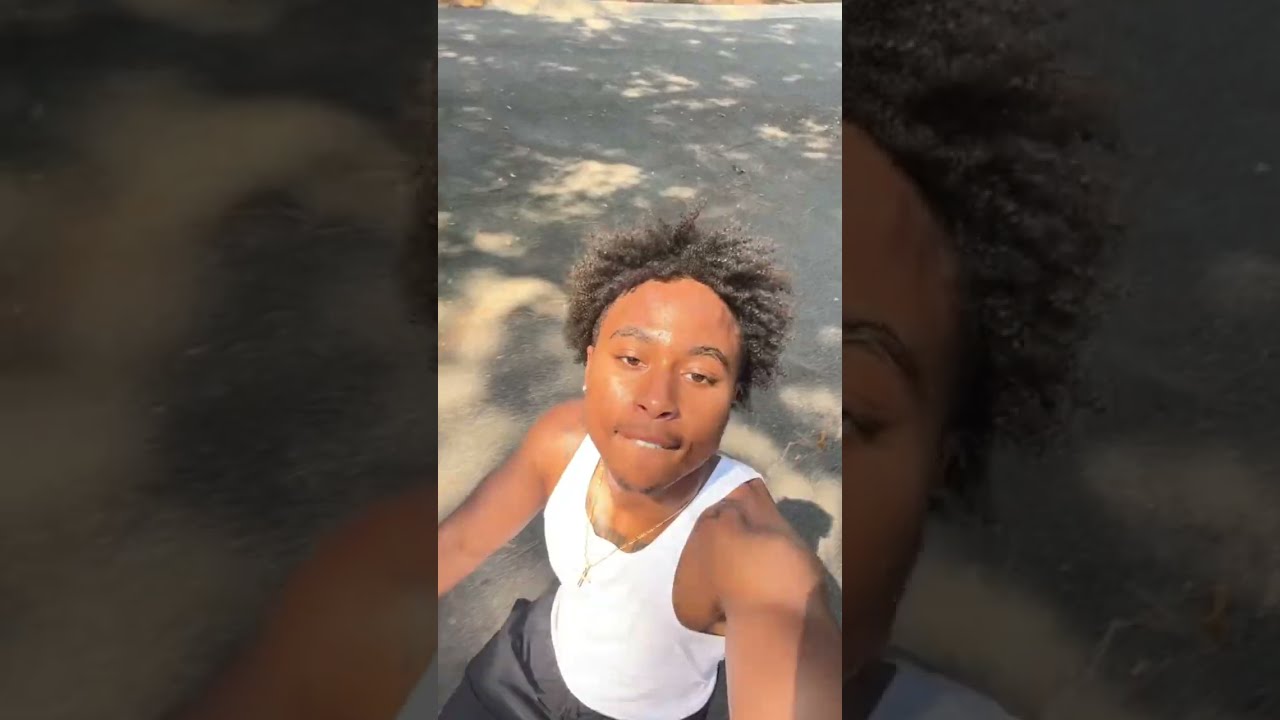The image features a muscular black man with a short, curly, nappy hairstyle, adorned with a thin mustache and some facial hair on his chin. He is taking a selfie outdoors, seemingly while riding a bike. His right arm is extended upward to hold the camera, capturing an angled shot of himself. He wears a snug white tank top, revealing tattoos underneath, and gray shorts that resemble basketball shorts. A gold chain with a cross dangles from his neck. The man bites his bottom lip, exposing his upper teeth. The background displays a gray, shaded, blacktop road, interspersed with patches of light and dark from tree shadows, as well as whitish rocks. Additionally, there are zoom-in sections to the left and right, showing close-ups of his arm, part of his curly hair, and face.